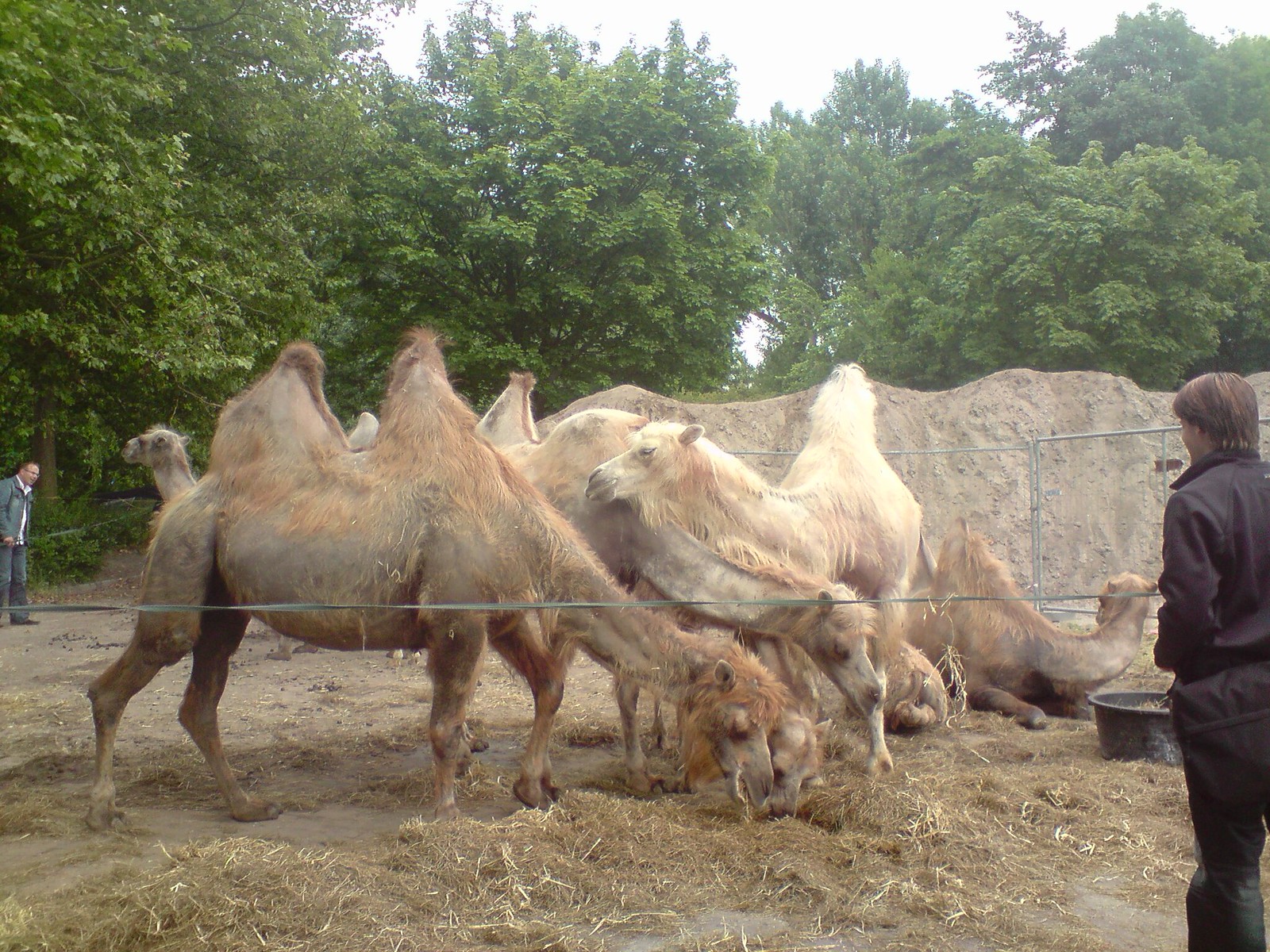In this outdoors photograph, we see six camels gathered in the center of a paddock, busy eating dry grass or hay from the ground. The camels, characterized by their sandy-colored hair and two humps, are enclosed by a single metal wire fence that stands at about human stomach height. To the right, a middle-aged man with medium-long black hair, wearing a black jacket and jeans, observes the camels. On the left, a second man, dressed in a grey jacket with a white shirt and grey jeans, also watches from a distance. The ground appears to be dirt-covered, scattered with hay, and a small black bucket is visible, possibly holding additional feed for the camels. The background is filled with green trees and a mound of dirt behind the metal fencing, under a white sky, indicating daytime.